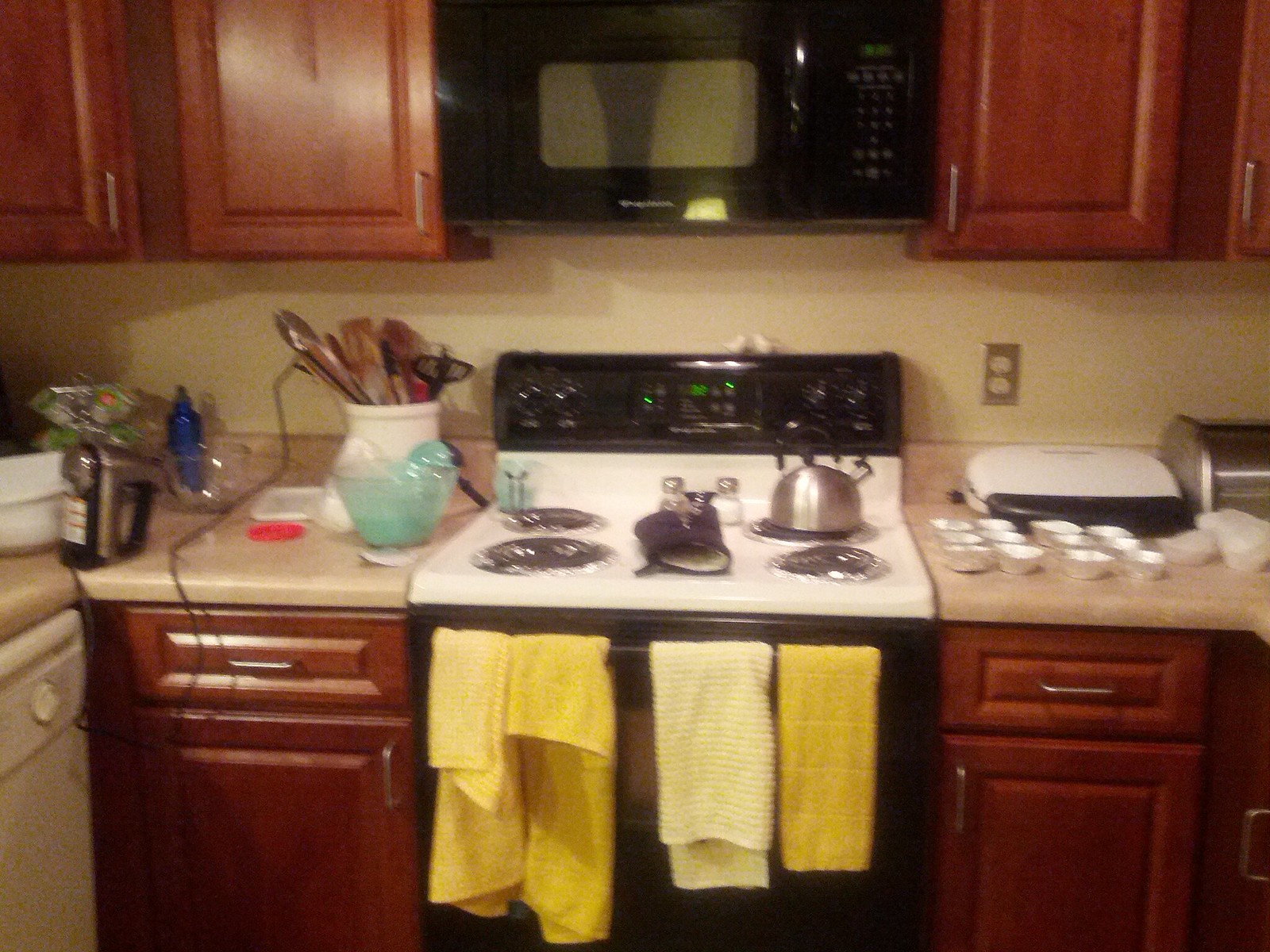The image depicts a nostalgic kitchen that appears to hail from the late 1980s or early 1990s, characterized by the grainy and slightly blurry quality of the photograph. The focal point of this kitchen is a large, central cooker featuring five rings on the hob. This black cooker has a white hob adorned with black rings, and the control knobs are located on a black panel at the top, which also houses a timer. Sitting atop the cooker is a kettle, complemented by a purple oven mitt and possibly some salt and pepper shakers.

The oven’s handle serves as a makeshift towel rack for four yellow and yellow-checked tea towels. Adjacent to the cooker, integrated into the cabinetry, is a black microwave. The kitchen cabinets themselves are a rich teak color, offering warm, reddish-brown tones and lining both the upper and lower sections of the wall we can see.

The countertops are cluttered with several kitchen essentials and appliances. Notably, there is a toastie maker, a set of bun cases, a bowl, and a utensil jar brimming with kitchen tools like wooden spoons and spatulas. An electric mixer, sans whisk attachment, sits among other indistinguishable items due to the image's blurriness. To the left, partially in view, stands a built-in white dishwasher or another large appliance, subtly blending into the room’s layout.

The scene captures a singular, well-used section of the kitchen, rich with the charm and details that define an era gone by.